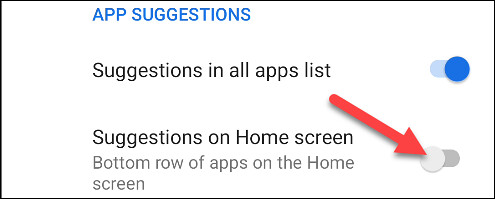The image showcases a mobile application interface screen, structured within a black rectangular frame and displayed on a white background. At the top of the screen, the text "App Suggestions" is prominently featured in blue. Beneath it, centrally located, is the option "Suggestions in All App Lists," which is marked with a blue check indicating activation. To the right of this option, the status is visually confirmed. Below, the text "Suggestions on Home Screen" is accompanied by a red arrow pointing downward towards an inactive toggle. This area highlights that the setting for "Bottom Row of Apps on the Home Screen" is not enabled.